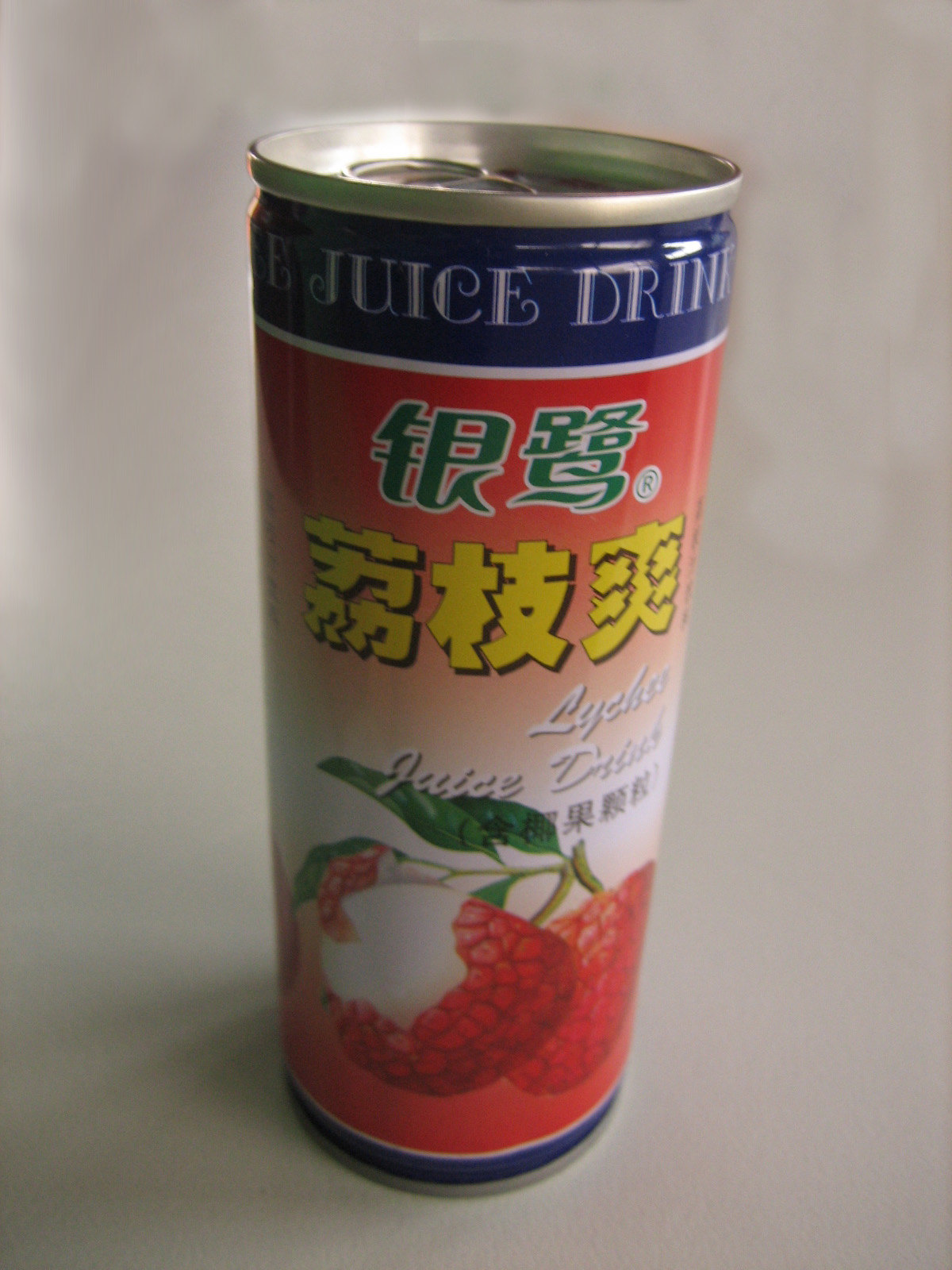In this image, we see a vertically standing canned drink with a distinctive design. At the very bottom of the can, there is a dark blue curved line that quickly transitions into a rich red color. The center of the can features a prominent illustration of a raspberry with a white filling in the middle and a green leaf above it. To the right of this illustration, there is white cursive text. The background color of the can changes from white to a faded red as it extends to the top. Near the top of the can, there is yellow text written in an Asian language, with green text in the same language placed above it. A white curved line is also visible near the top. Finally, the words "Juice Drink" are displayed in white text on a blue background at the very top, just below the silver, sealed top of the can. The entire scene is set against a light gray background.